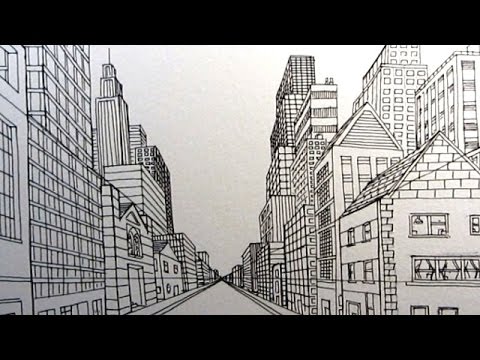This black and white cartoon-like drawing depicts a city street from the vantage point of someone standing at the beginning of the street, looking toward a vanishing point in the distance. The image is horizontally rectangular with black borders along the top and bottom. 

On either side of the street, sidewalks are visible. On the left, the buildings include a tall glass building, followed by a smaller two-story building with a gabled roof. Further along is a distinctive tall skyscraper resembling the Hancock Tower in Chicago, complete with a radio tower on top. Another glass and metal building precedes a smaller structure that appears distant due to perspective.

On the right side, a stone building with a gabled roof stands three stories tall, followed by a taller five-story building with a similar roofline. This side also features several narrower skyscrapers that are not as tall as the tower on the left. 

The street widens prominently at the bottom center and narrows to a pinpoint in the distance. The entire scene is devoid of text or people, focusing solely on the architectural elements and presenting an artist's interpretation of a cityscape.